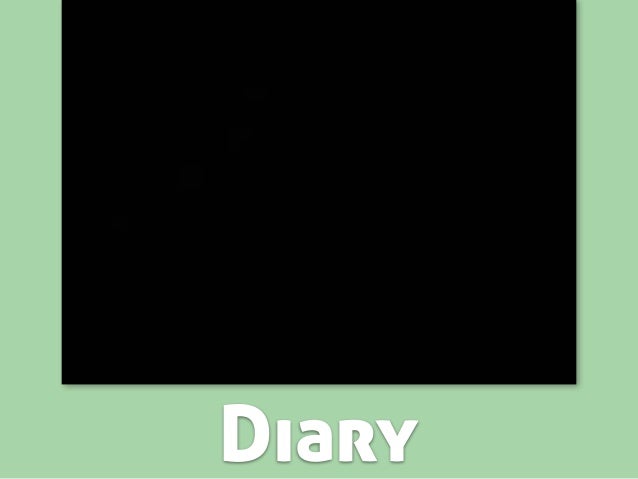The image depicts a largely digital or possibly drawn composition featuring a central black square with no content inside it. This black square serves as the focal point and is outlined by a mint green border on the left, right, and bottom sides. Positioned directly below the square is the word "DIARY" in all capitalized, bold white letters. The greenish background fills the remainder of the image, contributing to a minimalist and stark aesthetic. This could potentially be the front cover of an online journal or digital diary, characterized by its simplistic yet distinctive design.